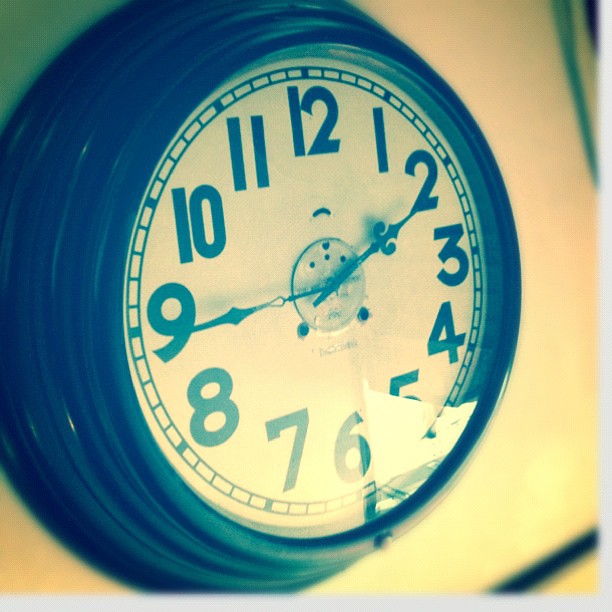This square, color-toned photograph features a prominently displayed wall clock, taking up two-thirds of the frame from left to right. The image has a distinct yellowish-peach cast, enhancing its vintage feel. The clock itself has a dark blue border, which is either metal or plastic, and a simple cream-colored face adorned with all twelve numerals in a straightforward design. The clock hands have an old-fashioned style with long, arrow-like points and a scroll base. The hands indicate the time is a quarter till two, with the short hand at the 2 and the long hand at the 9. At the center of the clock face, a circular metal disc secures the hands, flanked by two screws and an unreadable manufacturer's name. The background of the image is slightly blurred, featuring a light green wall in the upper left corner, and streaks of green and black in the upper and lower right corners respectively. The light source can be seen reflecting faintly at the bottom center of the clock, adding a subtle highlight to the overall scene.